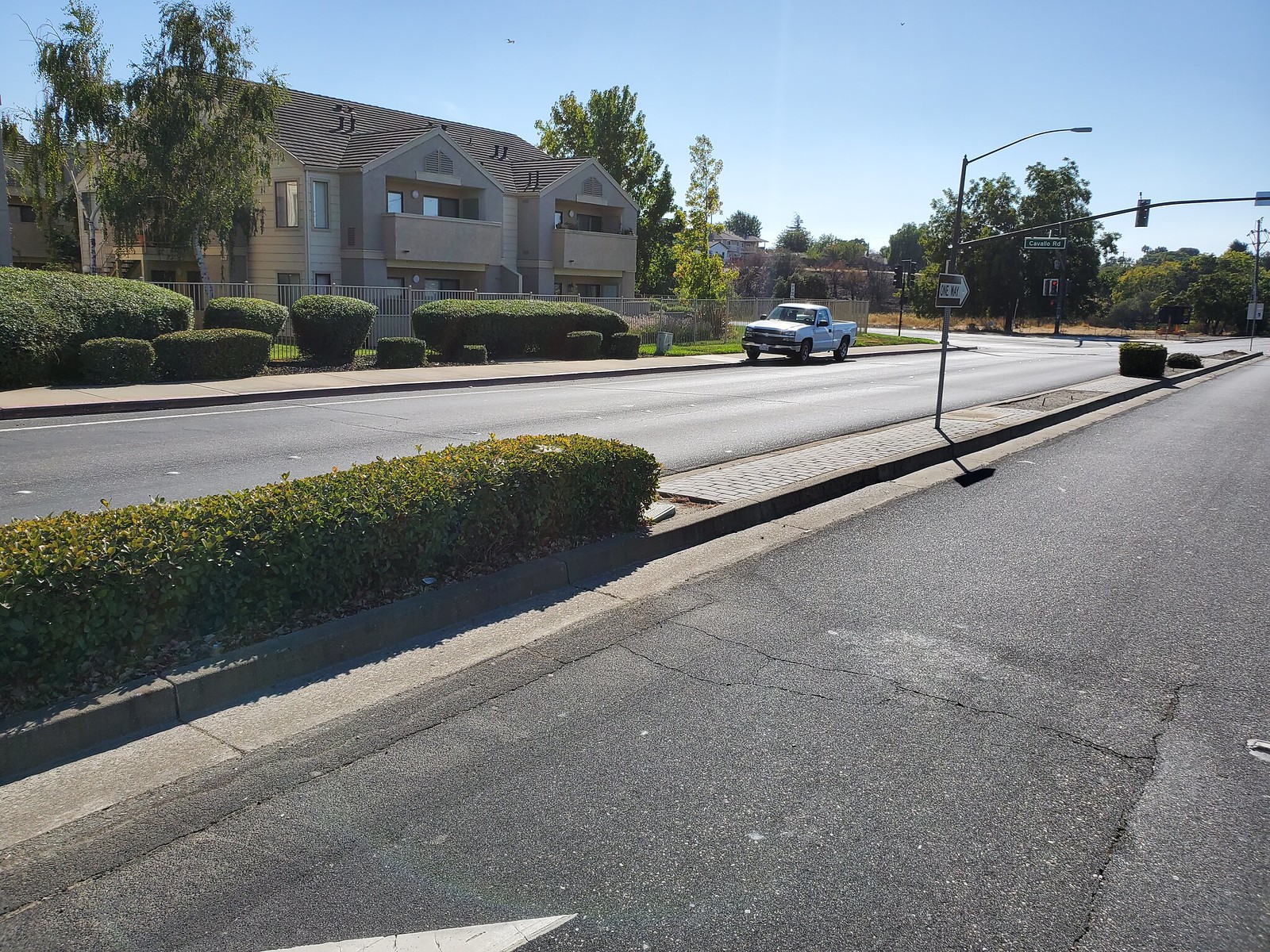In the image, a tranquil street extends into the distance under a vibrant blue sky that gradually lightens towards the horizon. On the left side, a charming house and what appears to be an apartment building stand amidst lush greenery, including trees and well-maintained hedges in front. A white pickup truck is parked along the curb, bordered by a neatly kept sidewalk. Further along the street, various hedges line the median, casting shadows that stretch across the concrete surface. A streetlight with an indistinct sign protrudes upwards, followed by a distant traffic light. There's also a glimpse of a white marking on the street, likely an arrow, though only a fragment is visible. Shadows from the hedges and streetlight add depth to the scene, capturing the peaceful ambiance of the neighborhood.